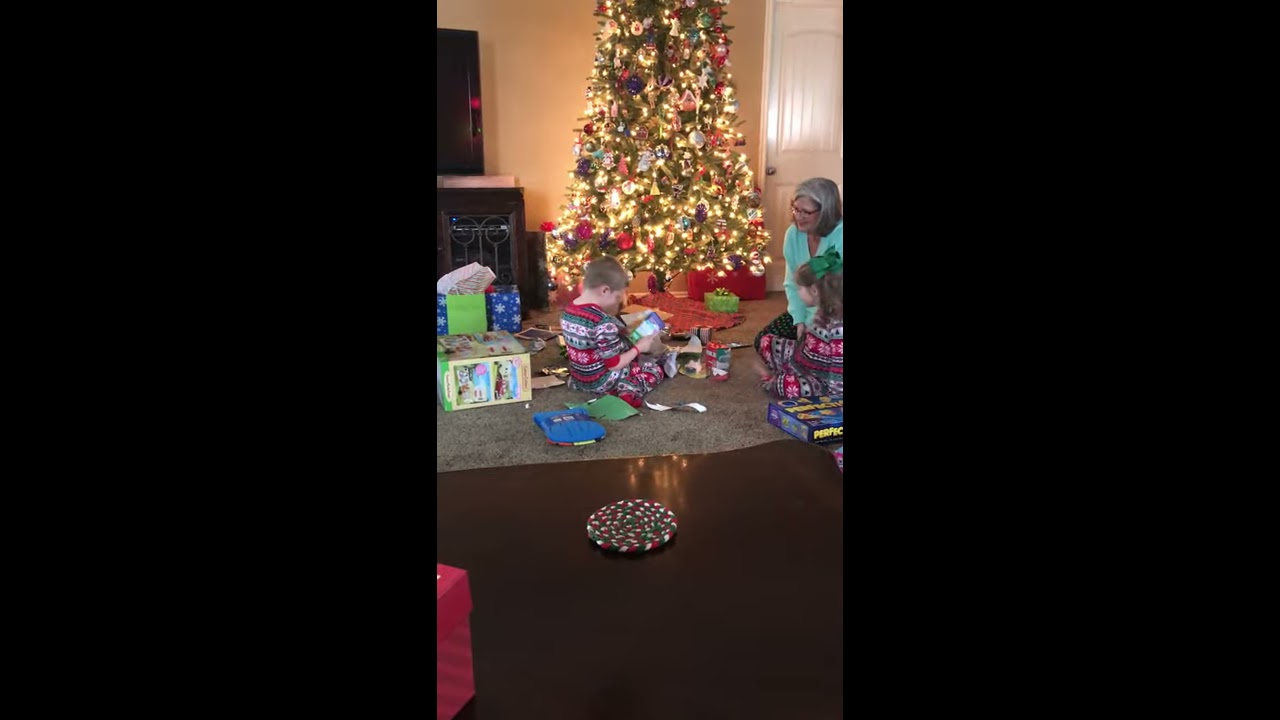This is a detailed photograph divided into three vertical panels. In the center panel, which captures the scene in portrait orientation, a festive Christmas setting unfolds. It shows three people seated on a grey carpeted floor. The carpet has a round pad in the center, and presents are scattered around, some already unwrapped. 

The room has cream-colored walls, with a white door on the right and a black cabinet partially visible on the left. A beautifully decorated Christmas tree adorned with numerous ornaments and twinkling yellow lights stands prominently in the background. The tree base is covered with a red plaid tree skirt, and a variety of colorful gifts, including a red present on the right, are placed underneath.

In the foreground, a young boy with short dark brown hair, dressed in festive red, green, and white pajamas, is enthusiastically opening a present. He is seated with his back slightly turned to the camera. To his right is an older woman, likely his grandmother, with shoulder-length salt-and-pepper hair, wearing glasses, a turquoise long-sleeve shirt with green dots, and dark pants. She watches the boy with a warm expression. Beside her and slightly in front of her is a young girl, possibly his sister, donned in matching holiday pajamas and a green bow in her long brown hair. She appears to be watching her brother intently. 

Toy boxes and other presents surround the children, indicative of the gift-sharing and festive atmosphere. The right and left panels of the image feature a solid black background, making the central Christmas scene pop with warmth and joyous activity.